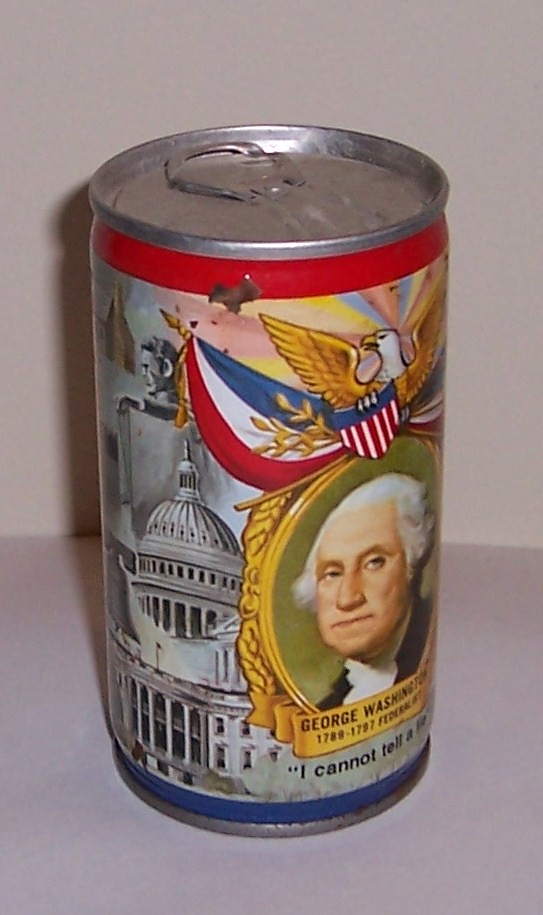The image features a vintage can adorned with historical and patriotic imagery. Prominently displayed on the can is a portrait of President George Washington, alongside an illustration of the United States Capitol building, an eagle, and the American flag. Additionally, there is an old side image of an unidentified person. Beneath Washington's portrait, the phrase "I cannot tell a lie," famously attributed to him, is inscribed. The top portion of the can is red, with the very top being silver and featuring an antiquated pull-tab design that is distinct from modern versions. The bottom of the can is also silver, with a blue strip just above it. The can is positioned on a gray table, set against a gray background.